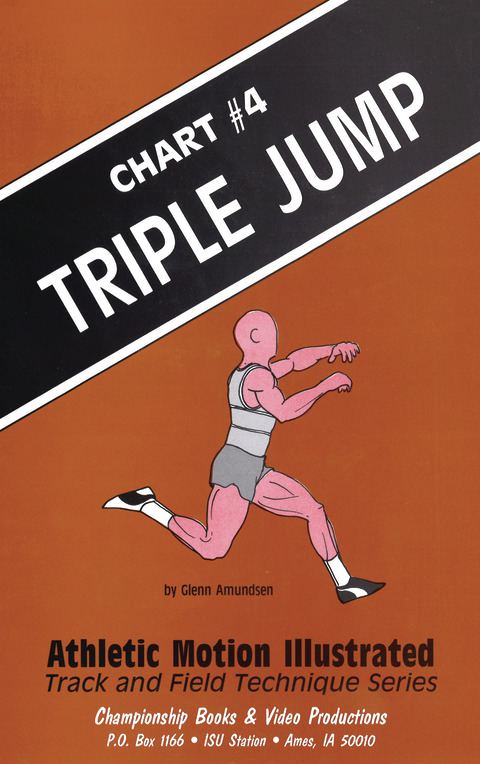This is a poster from a series in the Athletic Motion Illustrated Track and Field Technique Series. The background is a burnt orange umber, intersected by a black diagonal banner at the upper half, trimmed in white and featuring bold white text that reads, "Chart Number 4: Triple Jump." Below the banner is a stylized, almost crash test dummy-like illustration of a lean, muscular man in motion, wearing a gray tank top, shorts, white socks, and black and white tennis shoes, depicted mid-jump. At the bottom, it credits the author, Glenn Amundsen, and specifies the series' title. Further down, in white text, it reads, "Championship Books and Video Productions, P.O. Box 1166, ISU Station, Ames, IA 50010," suggesting it's part of an instructional exercise series.